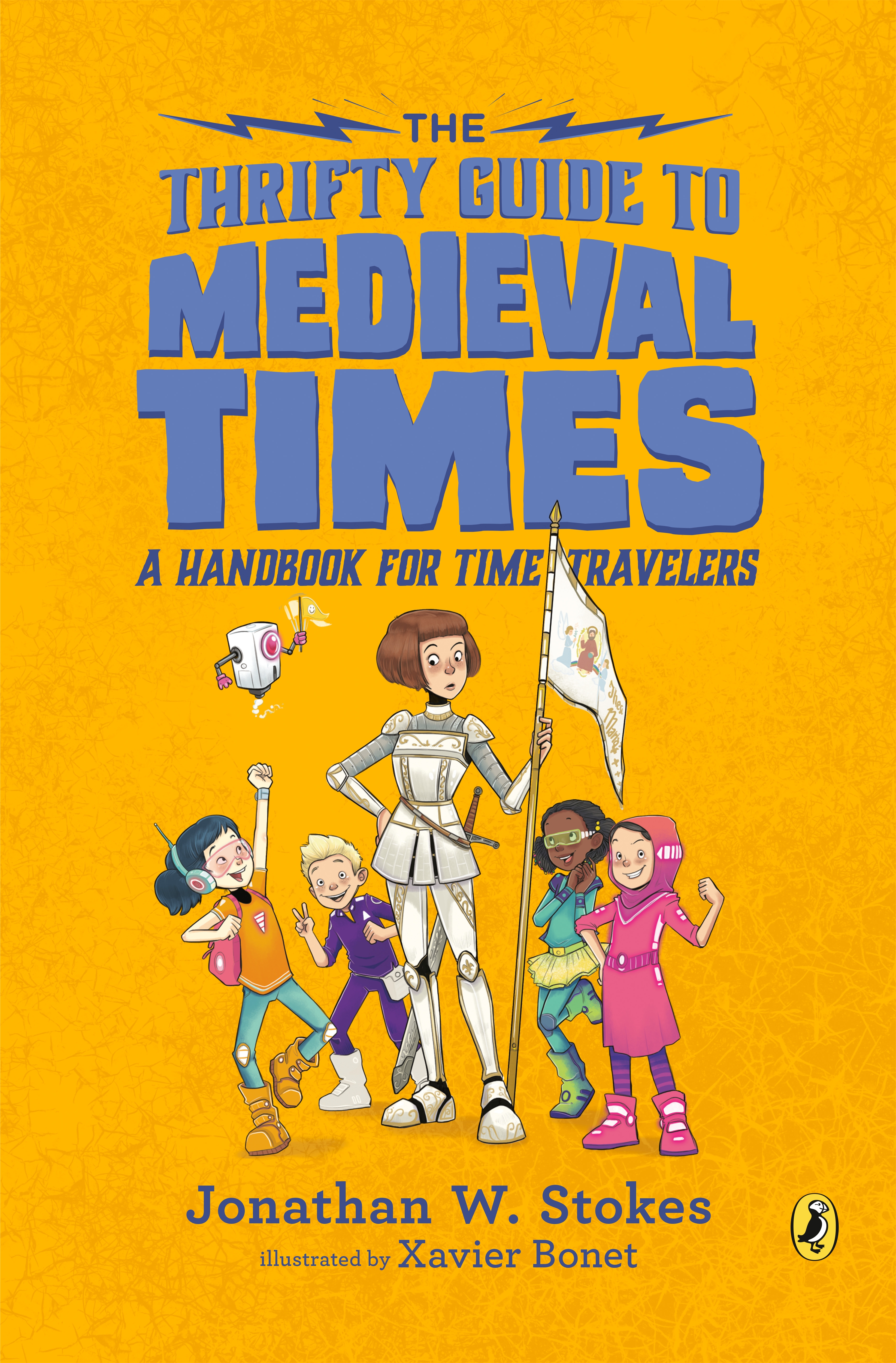This is the cover of the book "The Thrifty Guide to Medieval Times: A Handbook for Time Travelers" by Jonathan W. Stokes, illustrated by Xavier Bonet. The cover background is a vibrant orange with a marble-like grain texture. The title text at the top is formatted in dark blue, flanked by two lightning bolts, and the author and illustrator's names are at the bottom in the same color. In the illustration at the center, a woman resembling Joan of Arc, dressed in knight's armor with short brown hair and holding a silver and gray flag, stands prominently. Surrounding her are four children dressed in futuristic attire: to her left, a boy in a purple spacesuit and a girl with blue pants, a brown shirt, and headphones; to her right, a girl in a pink medieval outfit and a girl in a blue one. Additionally, there is a flying robot drone with a pointer hovering nearby on the left. A small penguin logo appears in an oval at the bottom right corner.